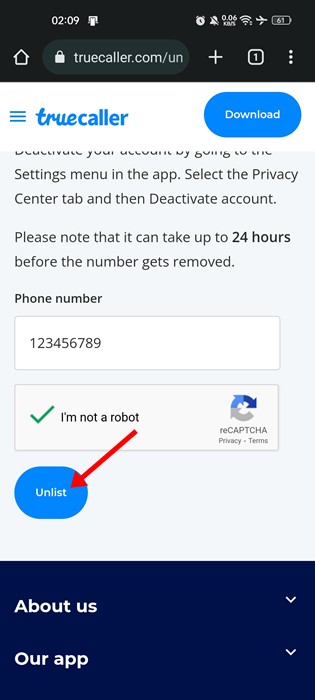This is a detailed screenshot of the Truecaller website taken from a mobile device. At the top left corner, there's a black status bar displaying the time as 2:09 in black text. The top right corner features several icons: an alarm symbol, a notification silence symbol, internet connectivity information, airplane mode, and a battery indicator showing 61% charge.

Beneath this status bar, there is the website heading "Truecaller" in blue against a white background. On the right side of this heading is a blue download button encased in a bubble. Just below these elements, there is a text box containing the phone number "123-456-789" and a reCAPTCHA verification that has a green checkmark signifying it has been completed.

A red arrow is pointing to a blue bubble that says “Unlist.” Further down, a navy blue bar labeled "About Us" in white text features a dropdown menu. Directly underneath this is another dropdown tab labeled "Our App." 

Overall, the image provides a comprehensive view of specific elements and navigational options available on the Truecaller mobile website.